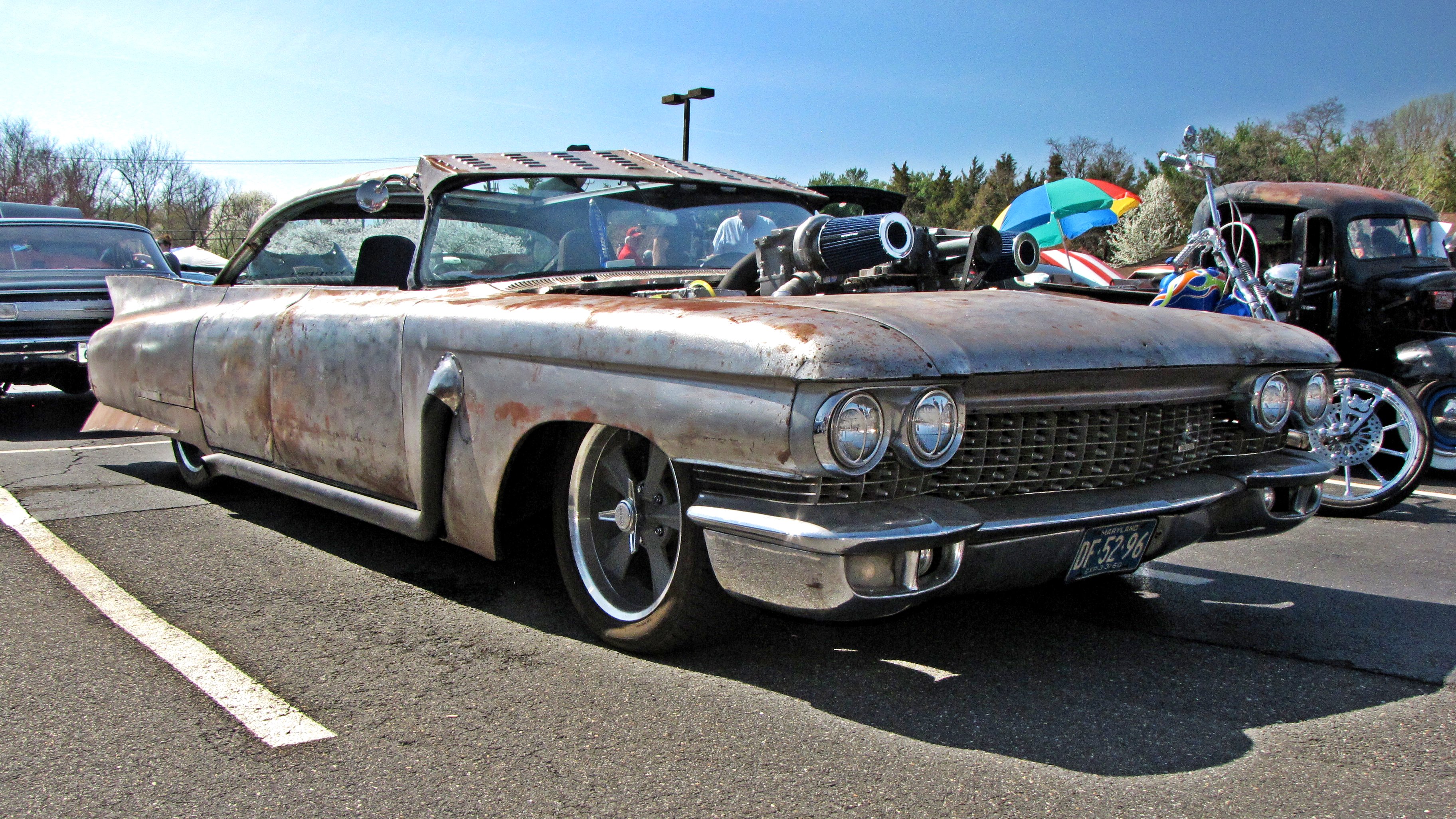A vibrant photograph captures a heavily modified early 1960s Cadillac Eldorado, taken outdoors during the daytime in landscape orientation. The viewer's perspective is from the front right diagonal, showcasing the vehicle’s distressed charm. The Cadillac's bodywork is extensively rusted, with patches of dark red and brown corrosion melding into a dull silver base, indicating a restoration project in progress. The paint has been stripped away, leaving the surface matte and unfinished.

Prominent modifications draw the eye; the hood features a significant cutout, revealing external twin turbochargers jutting out like formidable cannons, adding an aggressive, almost post-apocalyptic demeanor to the classic vehicle. The condition further reflects its journey through time— the lack of the middle pillar between the front and rear doors creates a striking open void along the car’s side, altering its original silhouette.

The front bumper hosts a rectangular license plate with a black background and white text, displaying the characters “D or O, F, 52, 96” in segmented formatting. This unique combination of elements provides a glimpse into the Cadillac’s past glory and its envisioned future, encapsulating a blend of history and mechanical ingenuity.